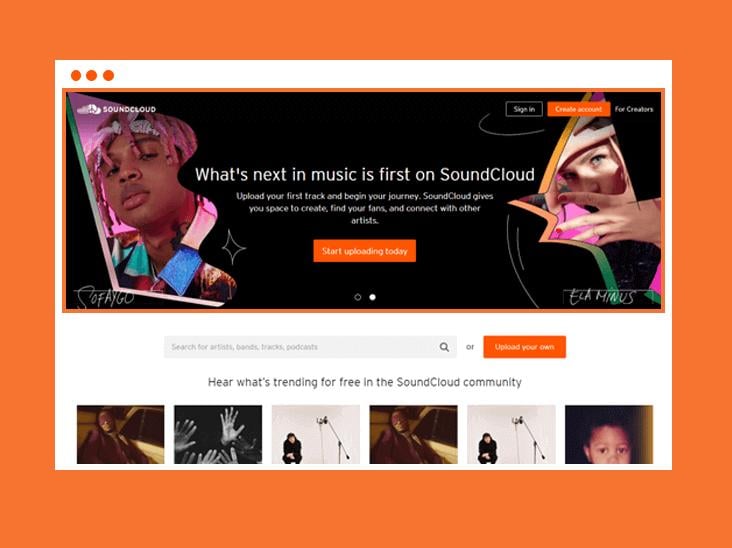A screenshot of the SoundCloud website is shown, highlighted with an orange border. The prominent banner across the top reads: "What's next in music is first on SoundCloud. Upload your first track and begin your journey." The banner emphasizes SoundCloud's role in providing a platform for creation, fan engagement, and artist connectivity. Below this message, a large orange rectangle button with white text invites users to "Start uploading today." The SoundCloud logo is situated in the upper left corner. 

Adjacent to the logo, there is a blurry search bar that prompts users to "Search for artists, bands, tracks, and podcasts," although the text is slightly unclear. Nearby, a section hinting at what is trending within the SoundCloud community can be seen. In the upper right corner, options to "Sign in" or "Create account" for creators are available. The overall layout suggests a user-friendly interface designed to encourage and support new artists in their musical journey.